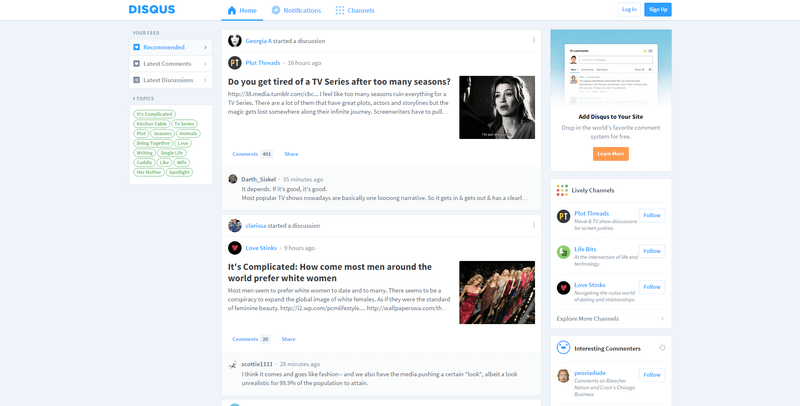This image displays the Disqus website interface. In the upper left corner, the Disqus logo is prominently featured. The top navigation bar includes various tabs such as Home, Notifications, and Channels, with the Home tab currently active. On the upper right side of the screen, there is a log-in or sign-up box, accompanied by additional clickable information. Below this, there is another section, possibly for learning more about the site or accessing specific features. To the right, smaller sections possibly showcasing news articles or site updates are visible. The main central area of the screen features images accompanying various posts or articles. On the left side, a sidebar provides navigational links for Recommendations, Latest Comments, and Latest Discussions, each indicated by accompanying arrows for further exploration.